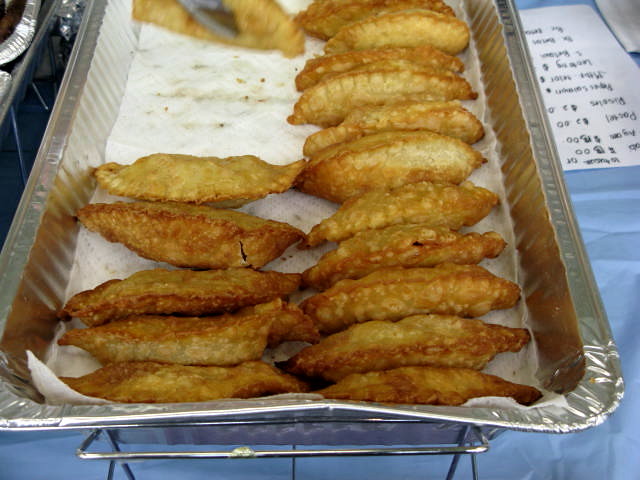This detailed image shows a central aluminum food tray filled with half-circle, oval-shaped pastries, likely empanadas or breaded items. The pastries are a golden-brown color and appear to be fried, resting on a white paper or cloth liner intended to absorb excess oil. The tray sits on a table covered with a blue tablecloth, suggesting a picnic or food stall setup. To the right of the tray, there's a piece of paper with handwritten details, probably listing prices or descriptions of the food items. Additional trays are partially visible on the left. The scene is illuminated in natural light, straddling the possibility of being indoors or outdoors.